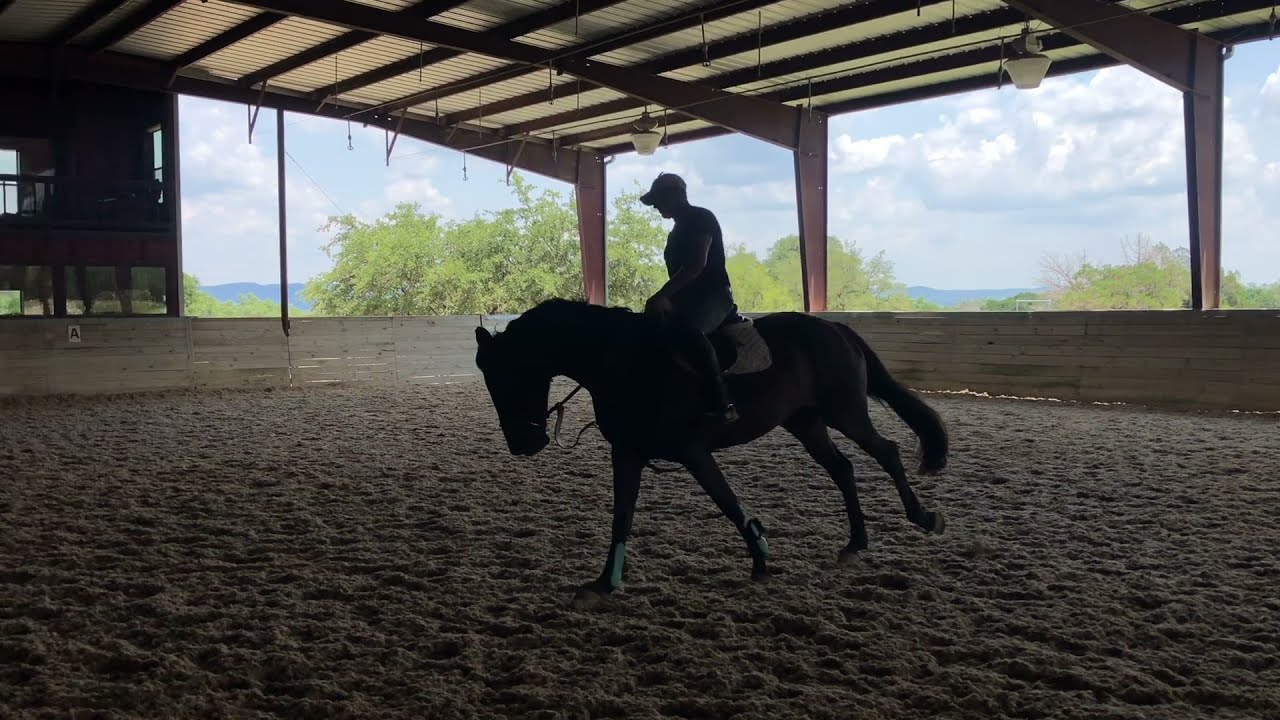In this horizontally aligned rectangular photograph, a man is riding a brown horse within a stable. The stable, with its short wood walls and ceiling canopy composed of variously aligned metal slats, creates a shadowy environment despite the bright, sunny conditions outside. The rider, wearing a dark baseball cap and indeterminate clothing, sits on a saddle as the horse prances on a sandy dirt ground marked by numerous footprints. The open sides of the stable reveal a backdrop of tall, green trees and a sky filled with white and gray puffy clouds. Although the interior is dark, the sunlight spills in from the sides, providing a stark contrast to the silhouette of the horse and rider.